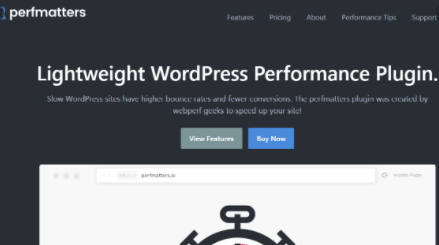A closely-cropped screenshot from the Perfmatters website features a sleek, user-friendly design with a dark gray to black background. The top navigation bar includes the Perfmatters logo on the left, followed by menu options for Features, Pricing, About, Performance Tips, and Support. The primary header text, presented in large white font, reads "Lightweight WordPress Performance Plugin." Beneath this, a subheading warns, "Slow WordPress sites have higher bounce rates and fewer conversions. The Perfmatters plugin was created by Web Perf Geeks to speed up your site."

Further down, two prominent buttons invite user interaction: a light green button with white text labeled "View Features," and a medium blue button with white text labeled "Buy Now." The image also includes a partially visible, large browser window showcasing the Perfmatters website's interface, incomplete but distinguishable by a black symbol on a light gray background.